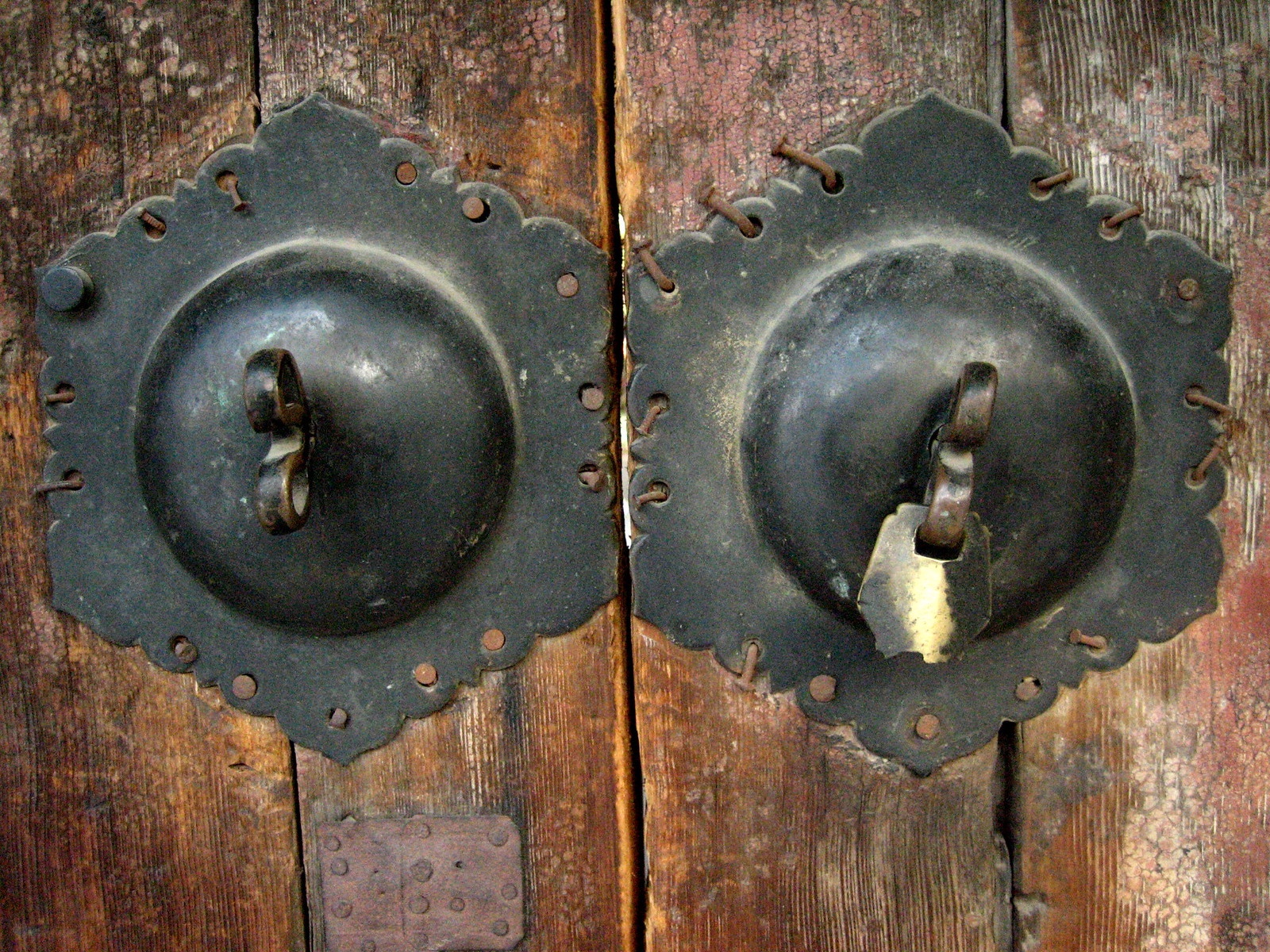This image is a close-up photograph of what appears to be an incredibly old and heavily weathered wooden door, featuring two intricate metal objects that might serve as door handles. The wood itself reveals extensive age and wear, with numerous cracks, marks, and chips. There's a notable mix of dark brown, beige, red, and lighter brown hues scattered across the wood. On the left side, particularly at the top, the wood showcases more beige and red tones, while the right side exhibits a progression from dark to more opaque brown, with chipping that uncovers white and red underneath. 

Both metal objects are similar in design, anchored at the center of the door. Each metal piece includes a raised, somewhat spherical circular section attached to a hexagonal backing. The metal on the left includes a black cylinder in the upper left, which is absent in the right object. On each of these raised circles is a wrought iron curly piece resembling the winding key of a clock, with two loops protruding from a protruding round shape of iron. The right object’s metal appears newer, perhaps better preserved, showing elements of steel with black on the right and white in the middle, surrounded by plain metal. Both objects feature a trapezoidal form with pitting and lines that seem like rusty nail marks, and a rivet on the left side. There's also a heart-shaped piece welded to the top with two small holes, with the right object having a metal piece extending out from one hole. Additionally, there’s a pink spot with gray circles in the lower left of the image, suggesting something was once attached but has since been removed or fallen off.